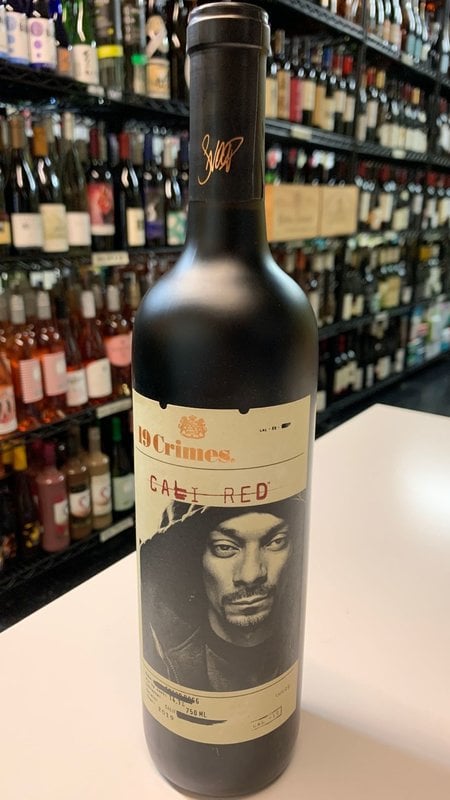This image captures a bottle of 19 Crimes Cali Red wine prominently displayed on a white counter, presumably in a liquor or wine store. The bottle is black and opaque with a cream-colored label that features a black-and-white image of the rapper Snoop Dogg, presumably Calvin Brodus. Snoop Dogg wears a hoodie and has a snarly expression. The label showcases the 19 Crimes brand name in gold lettering, with a crest or emblem also in gold near the top. The bottle is sealed, and a golden signature, presumably saying "Snoop," adorns the neck. Additional details like the wine being 750 milliliters are partially visible on the lower part of the label. In the background, there are shelves filled with various other bottles of wine and alcohol, though none are distinctly identifiable, keeping the focus on the featured bottle of 19 Crimes wine.